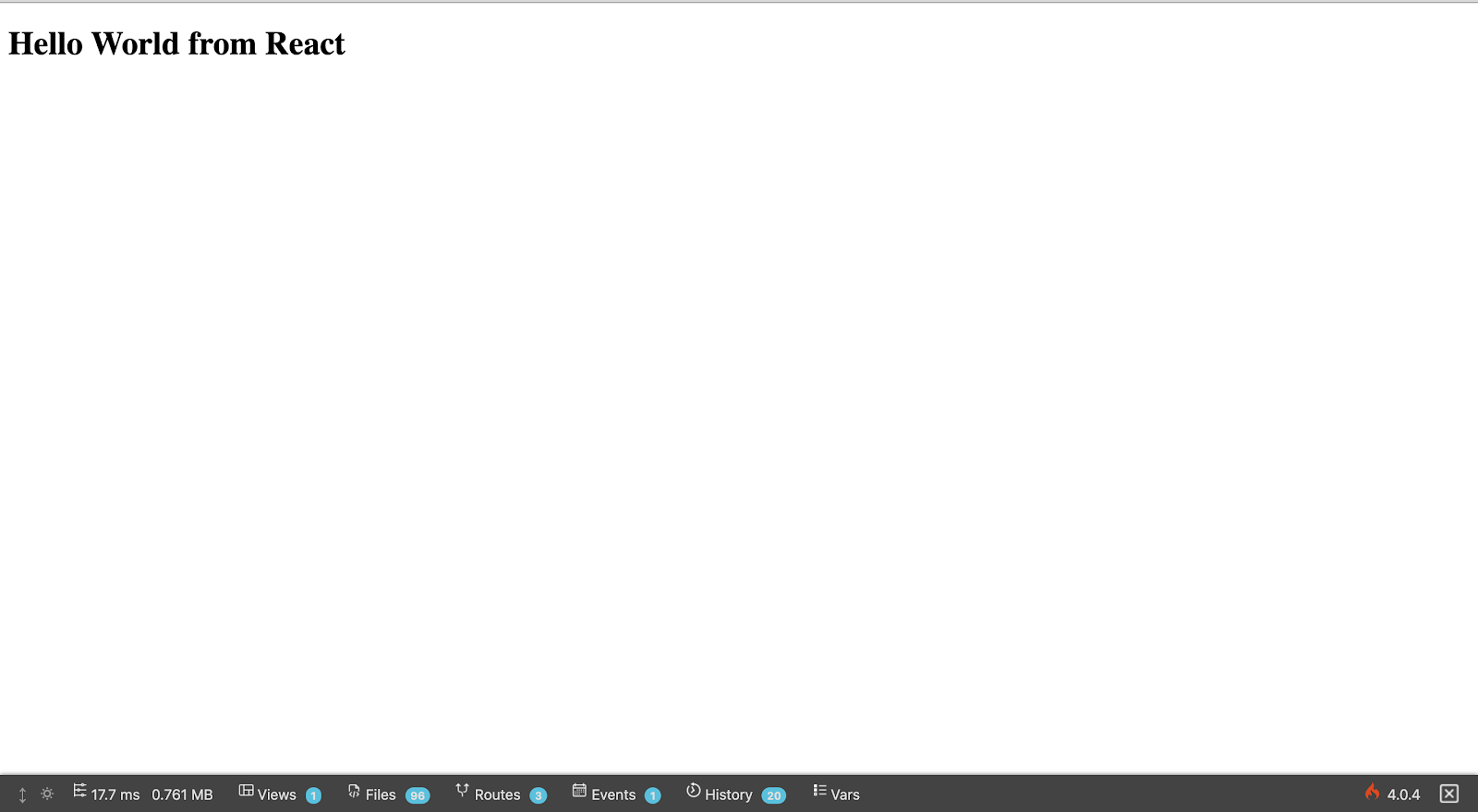This image is a screenshot of a minimalistic website potentially under development or encountering a loading issue, characterized by a stark white background with no visible content loaded. In the top left-hand corner, "Hello World from React" is prominently displayed in bold black font, though not overly large. In the bottom right-hand corner, a series of icons and text appears on a gray bar. A fire symbol is positioned next to the numbers "404", indicating a possible error. Along this gray bar, various interactive elements are shown: an up-and-down arrow, a sun icon, a side-to-side arrow, numerical values "17.7 ms" and "0.761 mb", and options to view "Views", "Files", "Routes", "Events", "History", and "Vars." The first five options are accompanied by blue icons, while "Vars" is denoted with a white hamburger-style menu. Toward the bottom right, adjacent to the 404 message and fire symbol, there's a white boxed "X" icon.